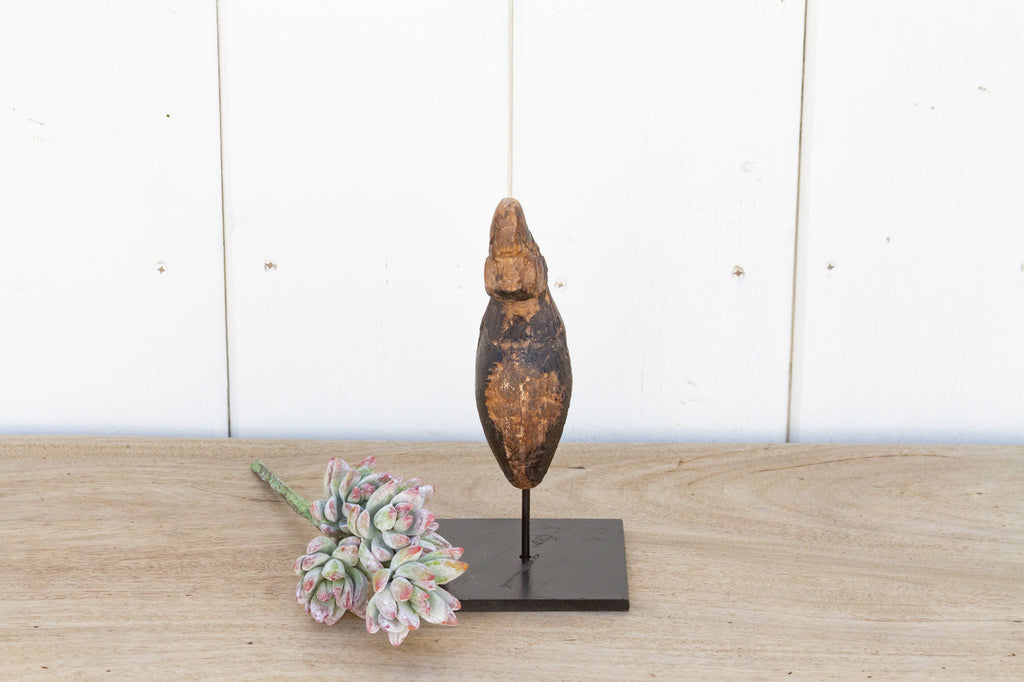The image features an enigmatic, carved wooden object, possibly antiquated, with an oblong, teardrop shape, mounted on a black stand. The object stands upright thanks to a central rod fixed to a square, flat base. This setup rests on a light-toned wooden surface, likely a table. Beside the wooden object lies a green and red succulent plant with frosty white tips, which may be faux, adding a vivid contrast. The backdrop consists of white planks, enhancing the brightness and clarity of the scene. Together, these elements create a visually intriguing composition, devoid of additional distractions.